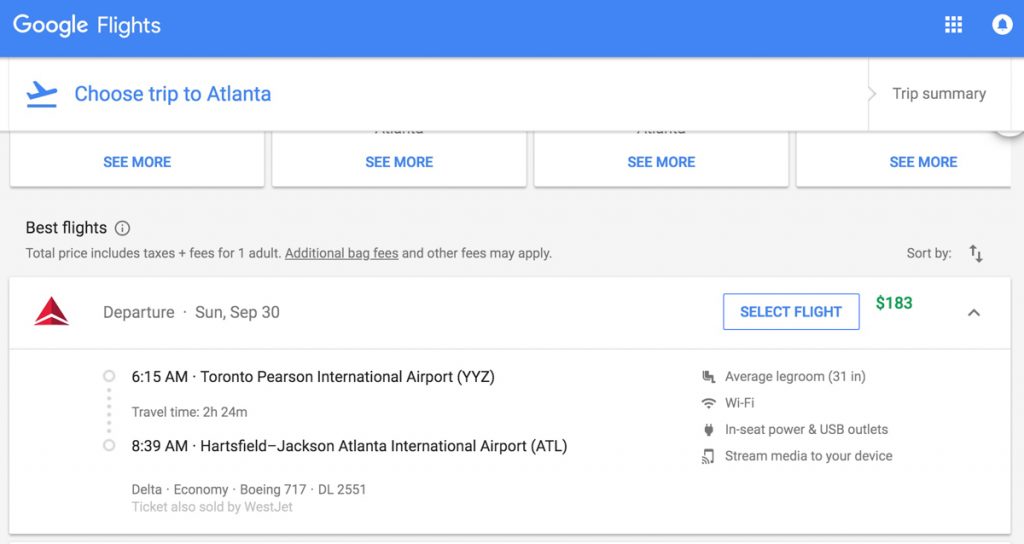This image is a detailed screenshot from the Google Flights website. At the top, there is a light blue and purple banner with "Google Flights" written in white on the left side. To the right of the banner, there is a white circle with a blue bell icon inside it. Additionally, three vertical white squares are positioned in a column.

Below the banner, the main body features a white background displaying flight information. Prominently, it states "Choose trip to Atlanta" with the option "Trip Summary" on the right side. Beneath this, there are four rectangular options, each labeled "See more."

Further down, a grey background section is titled "Best flights" and includes an information icon. This section clarifies that the total price includes taxes and fees for one adult, with additional bag fees and other charges potentially applying. An option to sort the results, marked with an "up and down arrow," is also present.

In the flight details area, details for a specific flight are provided: 
- Departure: September 30th at 6:15 AM from Toronto Pearson International Airport
- Travel time: 2 hours and 24 minutes
- Arrival: 8:39 AM at Hartsfield-Jackson Atlanta International Airport
- Airline: Delta Economy on a Boeing 717, also sold by WestJet
- Options: "Select flight" with a green $183 price tag

The flight information is visually supported by a red triangle icon adjacent to the departure details.